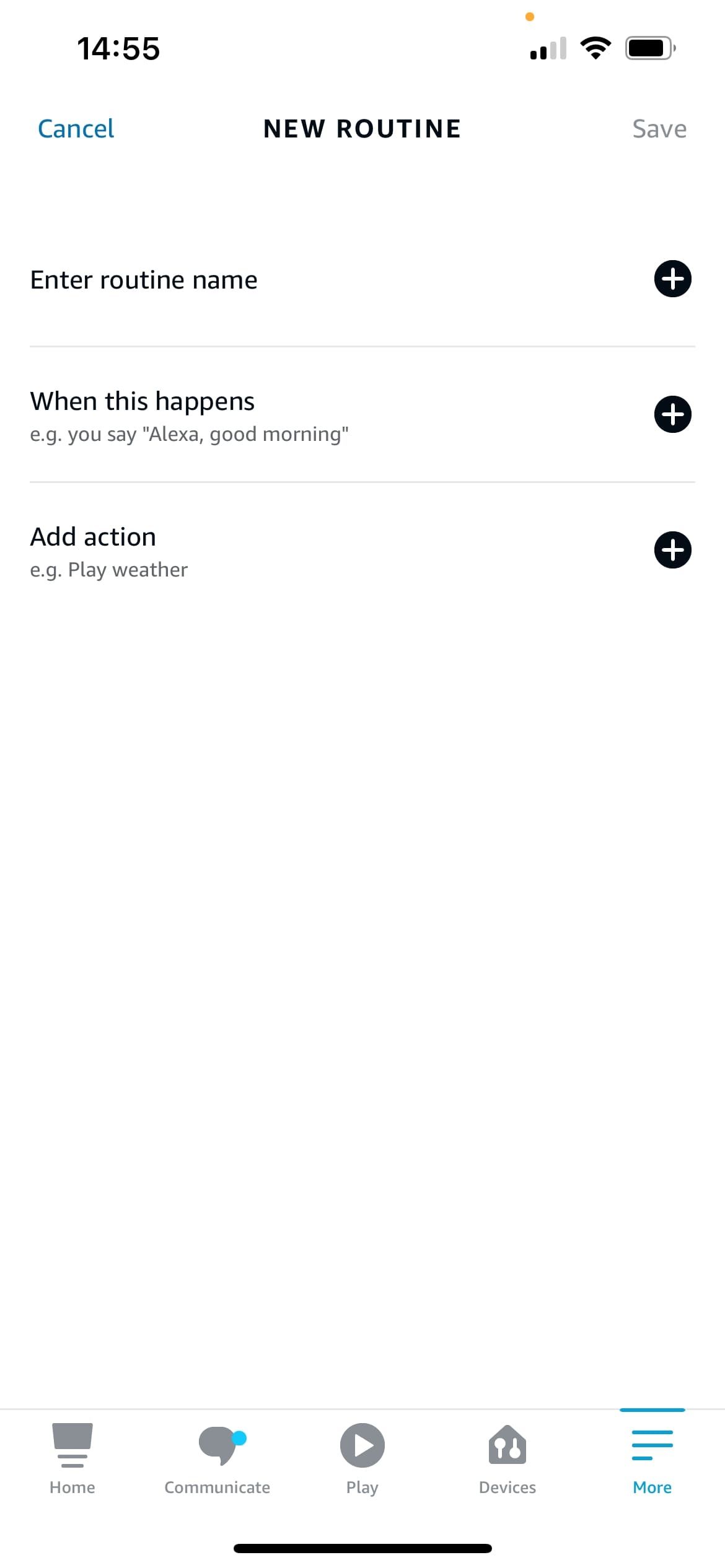The image depicts a user interface on a white background, illustrating the upper-left corner with a bolded, sans-serif font displaying "14:55." Adjacent to it on the right are signal strength bars, showing two out of four bars in black, with the remaining two in gray. On top of the first two bars is an orange dot. Further right, a fully black Wi-Fi signal icon is displayed, followed by a battery icon indicating about 80% charge with a partly filled black section.

Below this row, the interface continues with a "Cancel" option in blue on the left, and centered text in bold, spaced-out, capital letters reading "A NEW ROUTINE." To the right, in thin purple lettering, is the "Save" option. Directly under these options is an editable field labeled "Enter routine name" in black, with a gray underline indicating text can be inputted.

To the right of this field is a black filled-in circle with a white plus symbol inside. Below, in black text, it states "When this happens," followed by a gray example text, "e.g., you say 'Alexa, good morning'." To the right of this is another black filled-in circle with a white plus symbol, alongside a faint gray line.

Further down, the interface continues with a black text reading "Add action." Underneath, in gray text, it provides another example, "e.g., play weather." To the right of this text is yet another black filled-in circle with a white plus symbol in the center.